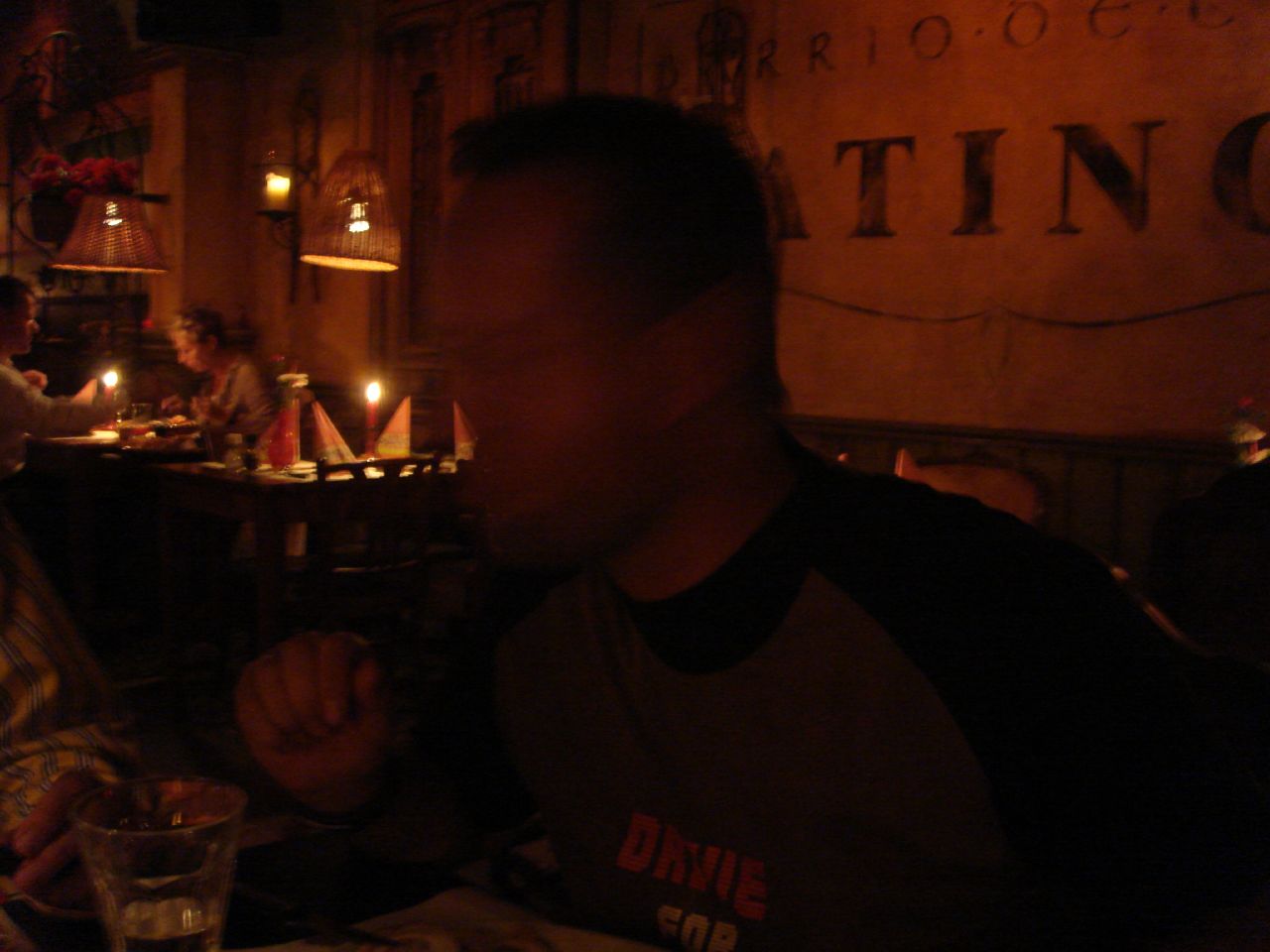The image shows a dimly-lit restaurant scene with a blurred person in the foreground, wearing a black and gray t-shirt that has partial lettering reading "Davey" in red and a yellow "4". The background features additional diners, including a couple seated together, creating a cozy atmosphere with tables adorned with candles and distinctive wicker basket hanging light fixtures. The blurred foreground figure is seated at the table with a glass, possibly containing water or alcohol, in front of him, and another person's left arm and hand partly visible. The restaurant's ambiance is enhanced by wall sconces and hanging flower baskets, and above the bar, there’s a large, partly obscured sign where the letters "T-I-N" are the most legible.